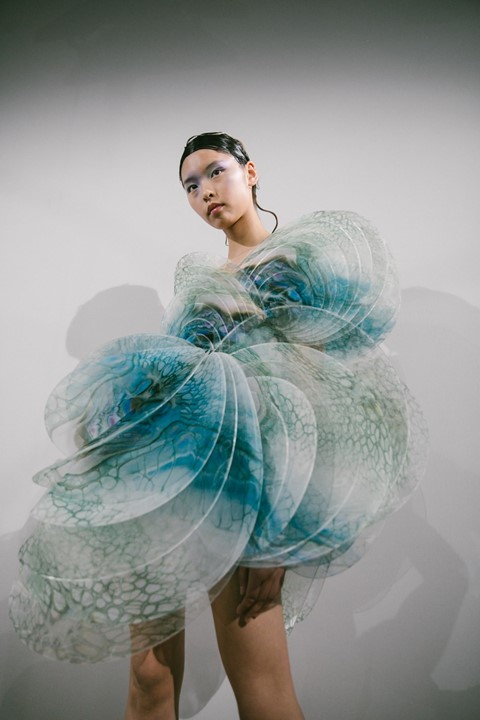This is an indoor color photograph of a young Asian female fashion model. The setting features a stark white backdrop that emphasizes the avant-garde nature of her attire. She appears to be in her late teens to early twenties, with slicked-back dark hair, giving her a sleek and polished look. Her head is slightly tilted to her right, her gaze directed towards someone behind the camera, and she has a serious, contemplative expression on her face.

A notable architectural touch is the dark gray streak across her eyes, which is more than an eye shadow, adding a dramatic flair to her appearance. Her dress, an abstract piece of high fashion, resembles a large, intricate flower or the folded wings of a butterfly. The dress is predominantly white with bold splashes of blue, creating an aquatic, ethereal effect. The short dress ends above her knees, constructed from layered circles of fabric, contributing to its unique, sculptural form.

The photograph is taken from a downward angle, capturing the model's form from her knees upward and casting her shadow on the plain backdrop. The overall composition, with the minimalist background and the striking outfit, turns the model into a living artwork, making this image a potential fit for a high-fashion magazine spread.